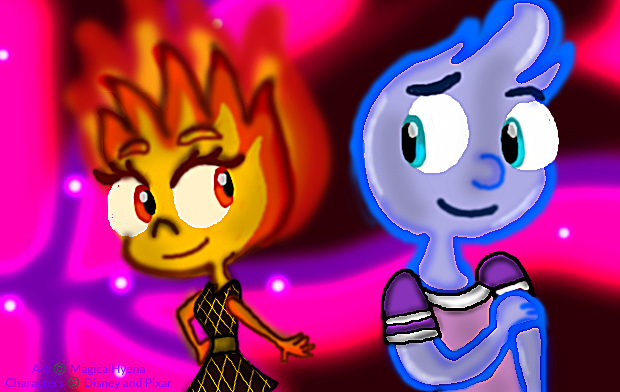The image is a detailed digital fan artwork, created by "Magical Hyena," featuring two characters inspired by Disney and Pixar's movie "Elemental." The background is a vibrant, almost neon pink, setting a vivid stage for the characters. The left side of the image showcases a female character with an orange and red flame head, complete with flames for hair and fiery red irises. She is dressed in a black, crosshatched triangle dress. To her right stands a male character, composed entirely of a blue, watery substance, with a rounded head topped by a watery crest. He is dressed in a pink shirt and stands with his back partially towards her, shyly rubbing his arm while glancing back. Both characters are smiling affectionately at each other, suggesting that they have a mutual crush. They appear close to each other, conveying a sense of intimacy and mutual interest, making this the focal point of the artwork.